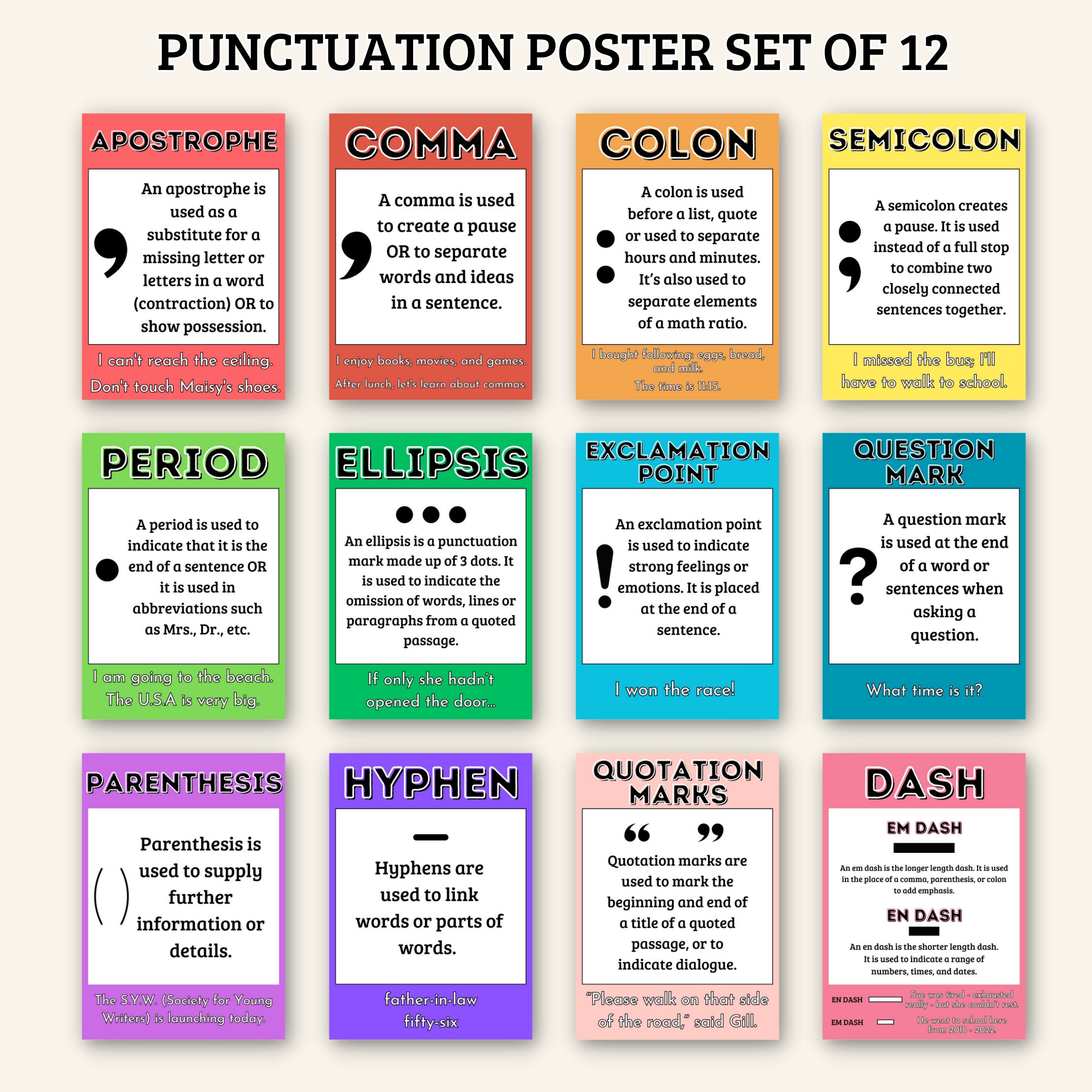The educational poster set, titled "Punctuation Poster Set of 12" in bold black letters at the top, features a comprehensive guide to punctuation. Arranged in a 4x3 grid with colored boxes, each poster focuses on a specific punctuation mark. The first row includes the Apostrophe (red), Comma (pink), Colon (orange), and Semicolon (yellow). The second row features the Period (green), Ellipsis (light green), Exclamation Point (blue), and Question Mark (dark blue). The third row displays Parentheses (purple), Hyphen (light purple), Quotation Marks (pink), and Dash (dark pink).

Each colored box contains the name of the punctuation mark at the top, the symbol in the center, and a detailed explanation of its usage. Additionally, there is an overlay of example sentences at the bottom of each box to illustrate the practical application of the punctuation mark. This detailed and visually organized poster set serves as an educational tool to instruct proper punctuation usage in writing.